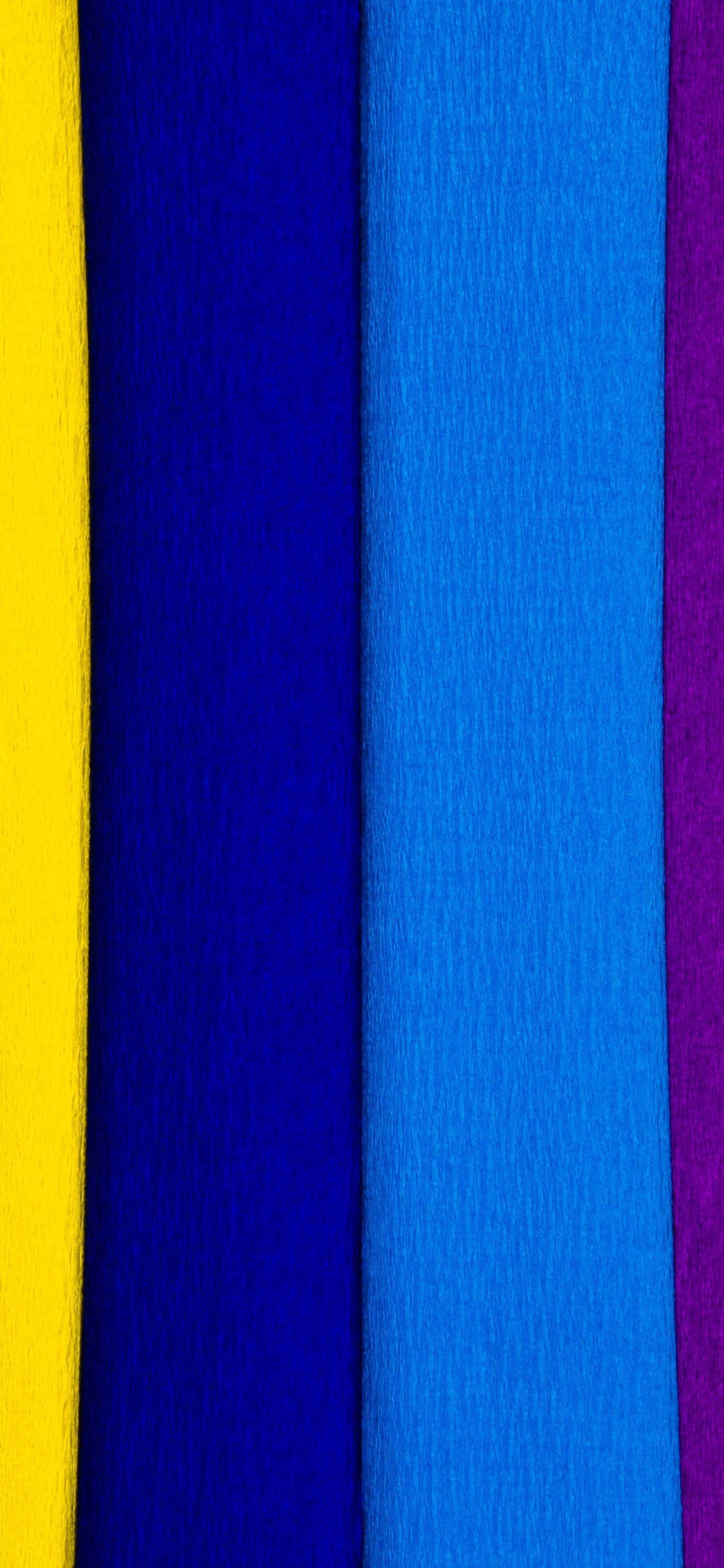This image is a tall and narrow portrait-style photograph, evidently longer than it is wide. The composition features four vertical bands of color resembling fabric or painted wood, possibly evoking the appearance of bolts of fabric on a shelf. From left to right, the colors are a bright yellow, a dark navy blue with a black border, a lighter sky blue, and a deep purple. The yellow and purple bands are thinner compared to the two blue bands, which are the thickest. All the bands exhibit a rough texture, hinting at materials like felt or towels. The leftmost and rightmost bands are partially cut off by the edges of the frame, further emphasizing the central bands in the overall composition.